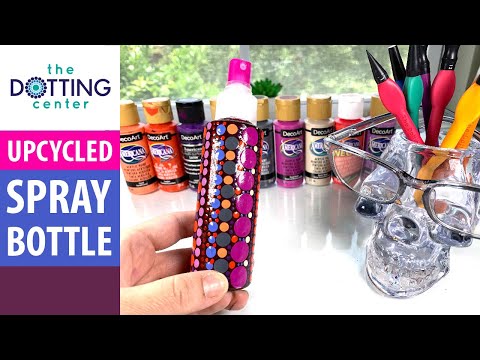The image appears to be an advertisement or a still from a video related to an arts and crafts business called "The Dotting Centre." It features a split layout with important informational text on the left and a detailed visual on the right. The header text on the left side is organized and colorful: the word "the" is in turquoise, "DOTTiNG" is in all caps dark navy text with an intricately spiraled "O," and "centre" is in turquoise. Below these headers are three strips: a pink rectangle with the word "upcycled" in white, a blue square stating "spray bottle" in white, and a burgundy rectangle.

On the right side of the image, the main visual depicts a crystal skull adorned with oversized glasses and serving as a holder for painting instruments with vibrant handles in red, turquoise, and yellow. In the forefront is a hand (partially off-screen) holding an ornately decorated spray bottle, featuring vertical stripes of purple and orange circles, a white ring near the top, and a pink nozzle facing the camera.

The background, set against a window revealing green foliage, showcases various bottled paints with gold flip caps in colors such as orange, purple, pink, silver, cream, and red. This display suggests a creative workspace, possibly at home, emphasizing the advertised "Upcycled Spray Bottle" amidst a lively and colorful setting.